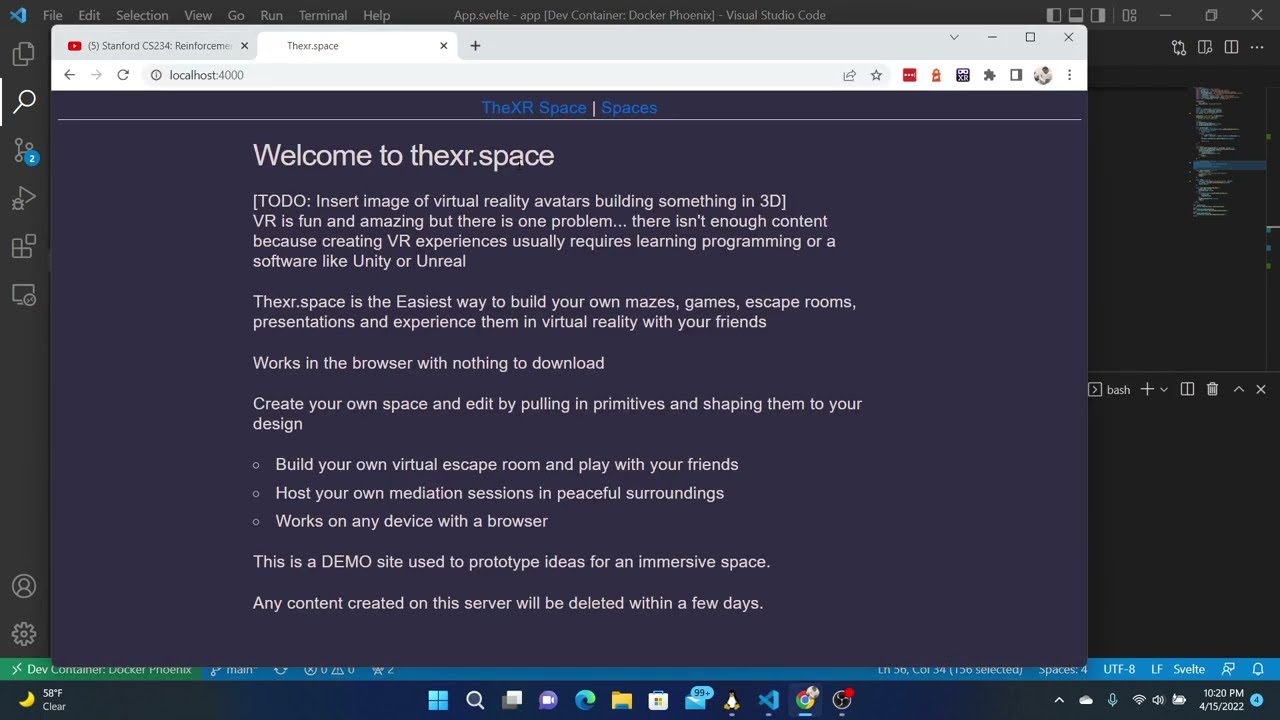The image is a screenshot of a computer display showing a web browser with two open tabs. The active tab's URL is "localhost:4000," displaying a web page titled "Welcome to the XR.space." The web page features detailed text against a purple background, highlighting the XR.space platform. It describes the site as an easy way to create virtual reality experiences, such as mazes, games, escape rooms, and meditation sessions, all within the browser without requiring downloads. Users can edit spaces by pulling in primitives and shaping them to their designs. Additionally, the site is presented as a demo for prototyping ideas for immersive spaces. The text includes phrases such as "insert image of virtual reality avatars building something in 3D" and mentions that VR is fun but often content-limited due to the need for programming knowledge. The browser window interface includes typical symbols like tabs, URL, and action icons, with a row of Windows system icons at the bottom right, showing the date, time, battery, Wi-Fi connection, and sound settings.